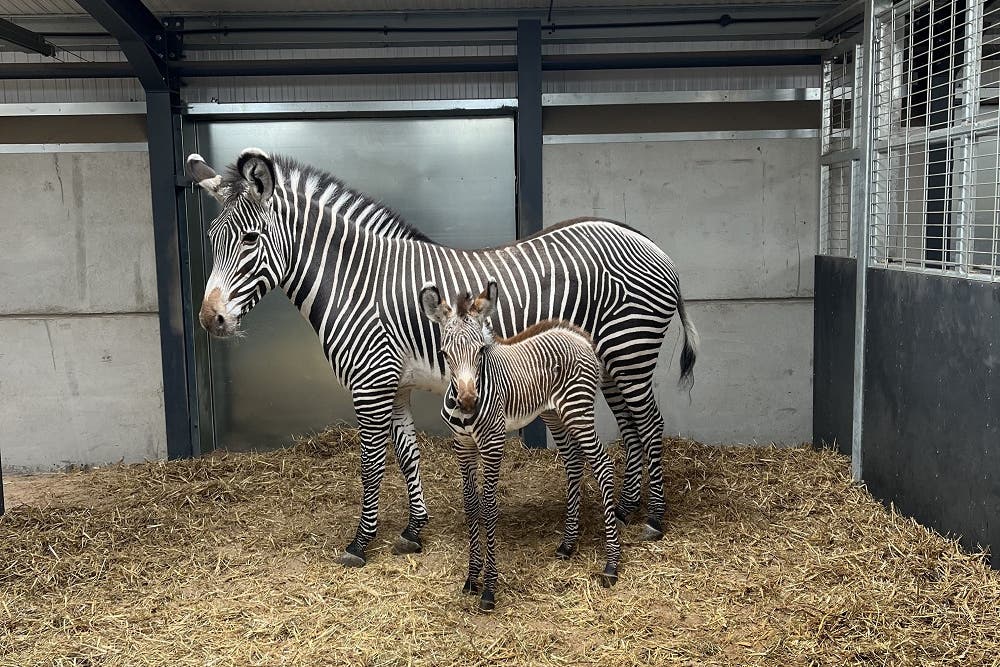In this captivating photo, an adult and a baby zebra are standing side by side in a modern, metallic stall with gray walls. The right side of the stall features a dark gray gate that offers a view beyond the stall. The floor is covered with straw, creating a natural bedding for the zebras. 

The mother zebra stands in a slightly sideways profile with her head turned to the left, her face angled slightly towards the camera. Her classic black and white stripes extend down her mane, and her ears are marked with a striking pattern of white and black on the inside. Her eyes are dark and expressive, and her nose transitions from a solid white to a delicate pink before turning black at her nostrils. Her sturdy hooves are gray with touches of black.

In front of her stands the adorable baby zebra, looking directly into the camera with an endearing gaze. Unlike his mother, the baby has a hint of brown in his short mane, which runs down the length of his back. His coat features the characteristic bold black and white stripes, but his nose and the top of his head display a soft brown hue, adding a unique touch to his appearance. Both zebras exude an elegant beauty, captured perfectly in this detailed and heartwarming moment.